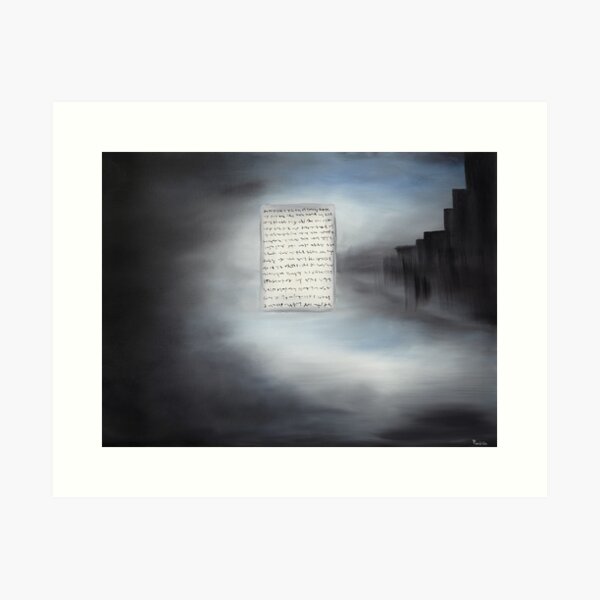The artwork, framed in a simple white frame, depicts a moody and atmospheric scene where dark, stormy clouds transition from black to grey, creating a haunting background. Central to the piece is a piece of paper with rows of small, illegible handwriting, surrounded by a thin white mist that contrasts with the darker surroundings. On either side of the paper, vague forms of stone pillars or structures can be discerned, adding to the enigmatic feel of the image. The sky to the right of the paper reveals a subtle hint of blue, breaking through the otherwise ominous cloud cover. Further scrutiny reveals a barely visible watermark in the bottom right-hand corner, adding an additional layer of mystery to the artwork.